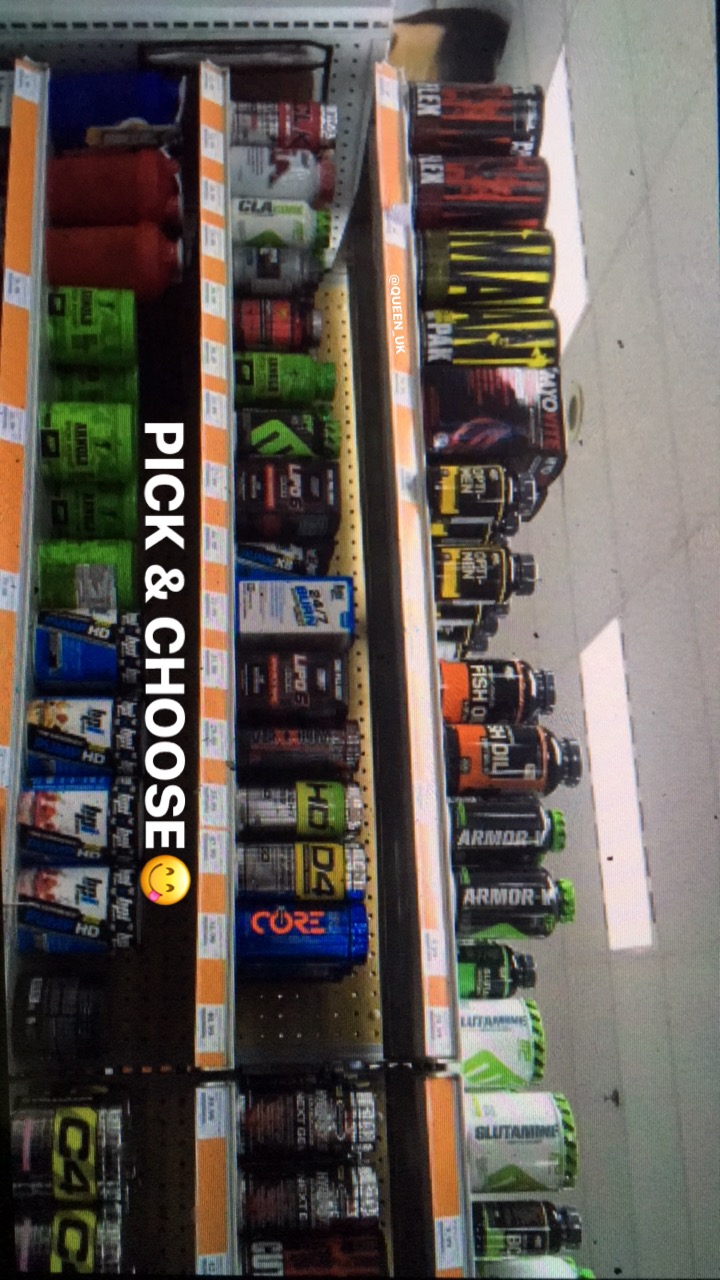This image, oriented vertically, depicts shelves in a supplements aisle of a store, turned sideways. The shelves are packed with various energy and protein powder containers along with some energy drinks, which come in vibrant colors including yellow, black, green, red, blue, and orange. The labels visible on these products include brand names like C4, Core, Armor, Glutamine, and CLA. An overlay text, reading "Pick and Choose," with a smiling emoji featuring a tongue sticking out, adorns the image. The shelves have distinct orange and white price tags beneath the items. The ceiling, visible in the image, consists of white panels and large LED lights. There is also a watermark in the lower portion, reading "@Queen_UK".